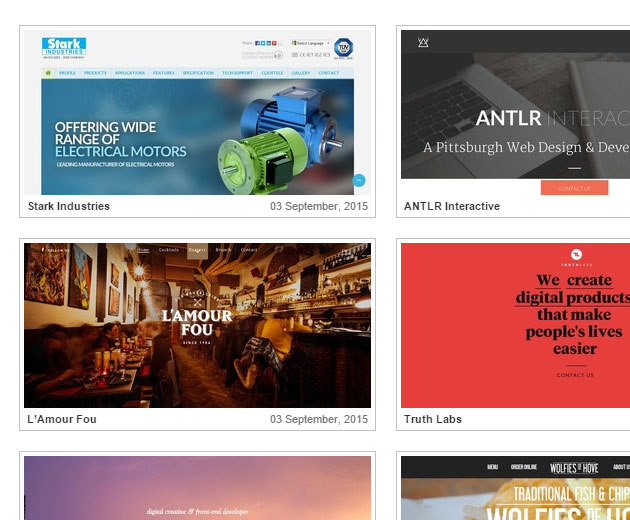This square screenshot captures a meticulously arranged grid of various box-like segments, each bordered by a thin grey line. The segments feature an assorted range of company images and text snippets, each providing a glimpse into the respective webpage designs.

On the left-hand section, two complete rectangular boxes are visible. The first box displays the homepage of Stark Industries, marked at the bottom left with the label "Stark Industries" and dated "3rd September 2015" on the bottom right in black text. The Stark Industries homepage has a dominant blue theme, showcasing their blue and white logo at the top. Centrally placed is an image of a piece of equipment, beside which is the text "offering a range of" in white, followed by "electrical motors" in blue.

Below this, within another thin grey-bordered box, is the company L'Amour Fou, also dated "3rd September 2015". At the center of this box is the white text "L'Amour Fou." The background features a blurred image of a bustling bar with an orange filter, displaying the bar front to the right and patrons at tables on the left.

To the right, two vertically stacked boxes appear partially cut off by the image's right border. The top box pertains to ANTLR Interactive, showcasing a heavily grey-toned background with "ANTLR" in prominent white text, followed by partially cut-off grey text "INTERACT". Below this, in white, reads "Epicsburg, Web Design and DEVERE", which is also truncated.

The box beneath ANTLR Interactive belongs to Truth Labs. It possesses a solid reddish-pink background, featuring black text near the image's right edge stating, "We create digital projects that make people's lives easier."

Shifting focus to the bottom, two boxes are clipped by the image's lower border. The bottom left box, only partially visible, transitions from dark purple to light purple, then pink to yellow from left to right. 

In the bottom right box, the top of another company's webpage is visible, including a black bar with white text saying "WOLF" and "HOME." The underlying webpage reveals a partially visible phrase "Traditional Fish and Chip," with the word "WOLFS" seen further down. The background includes a faint view of the sky and food items, though they are partly obscured.

This detailed and structured screenshot provides an intricate look at various corporate web designs and aesthetics, meticulously capturing the essence of each represented company.